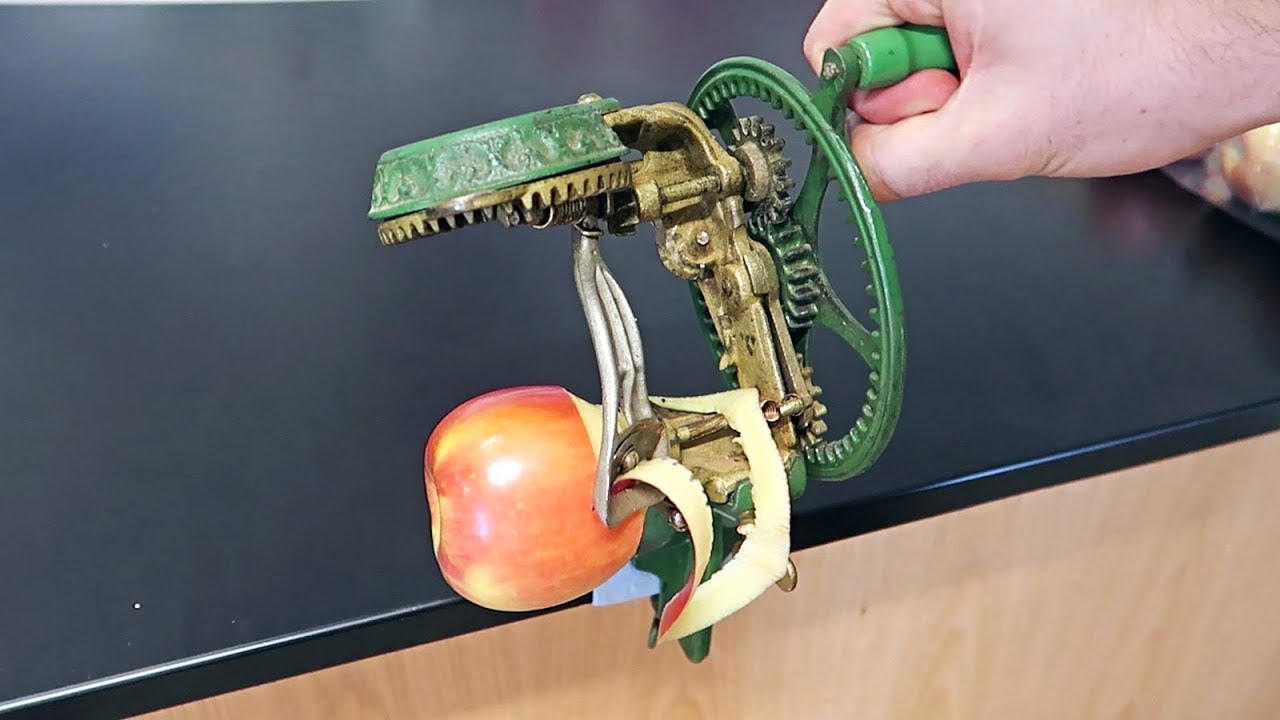The image depicts a horizontal, archangular antique apple peeler in use. A person is cranking the device with their right hand, turning a green wheel attached to the mechanism. This wheel, connected to a brownish beige-green metallic structure in the center, features a blade that presses against the apple. The apple is mounted sideways on the left side of the device; as the crank turns, the blade expertly slides underneath the apple's skin, peeling it. The device also includes a prominent gear-like component that holds the wheel and a green disc at the top that likely secures the blade's position against the apple. The apple peel is visibly accumulating as it is removed. The scene is set on a black, shiny countertop with a wooden base, suggesting it's in a kitchen environment.